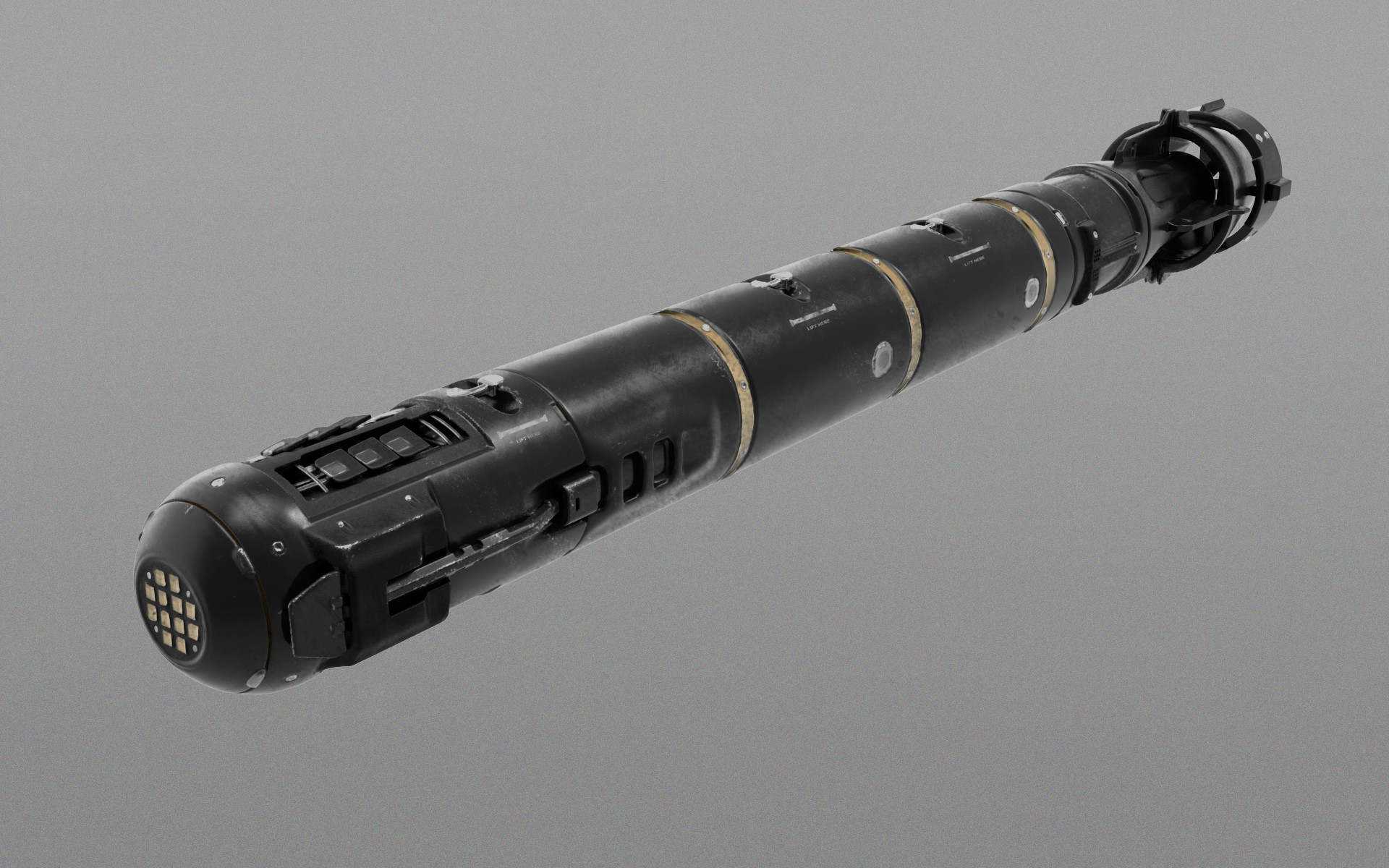The image depicts a long, cylindrical black object with a metallic sheen, resting on a gray background. The object, which resembles a ballistic missile or possibly a torpedo, has a front end featuring a grating with gold-colored material inside. The body is segmented, with several black sections separated by gold stripes. The object's top and bottom surfaces are flat, with the upper area displaying what might be buttons or lights, indicative of potential control mechanisms. The rear end presents a double-ring structure that could be an encased propeller or turbine, suggesting a capability for underwater movement. The front, pointing down towards the bottom left corner, has a circular screen composed of small square patterns, hinting at sensor or light apparatus.